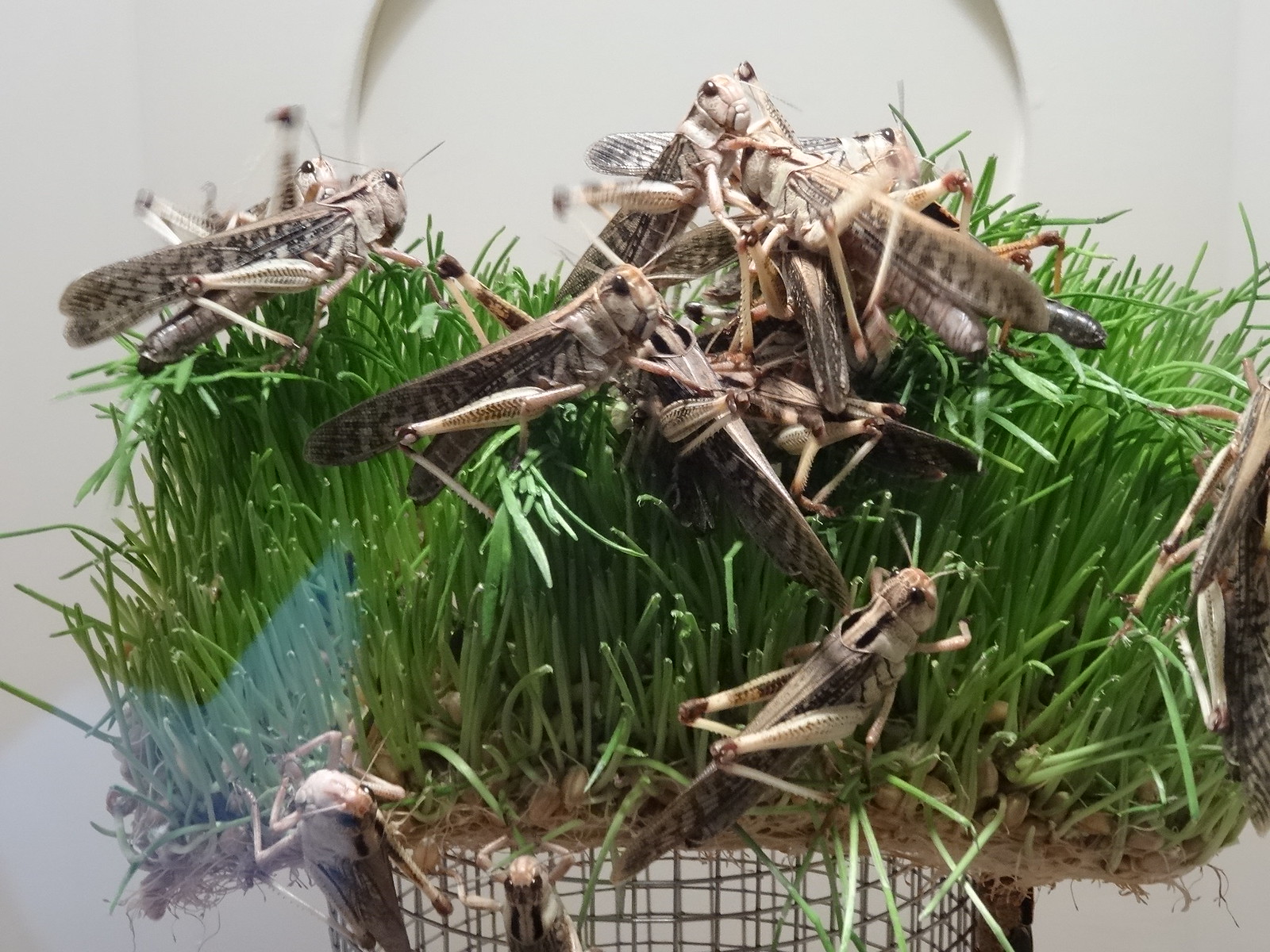The image depicts a multitude of large brown grasshoppers congregating on a cube of artificial green grass that appears to be set within a cage-like structure or basket. The grass, akin to fake astroturf, is placed on top of a metal framework with a beige handle partially visible at the top. The background is a featureless, blurry white, drawing attention to the vividly detailed grasshoppers. These insects, possibly mistaken initially for moths or cicadas due to their beige and dark brown coloration, are shown in various states of motion, with some climbing up the cage and others stationary, leading to occasional motion blur. The image is sharply lit from above, highlighting the rubbery texture of the grasshoppers' bodies, the barbs on their feet, their spindly legs, and the intricate details of their wings. The composition is meticulously focused, allowing an up-close view of the insects’ anatomy, including their beady eyes and antennae, set against the stark contrast of the artificial greenery.